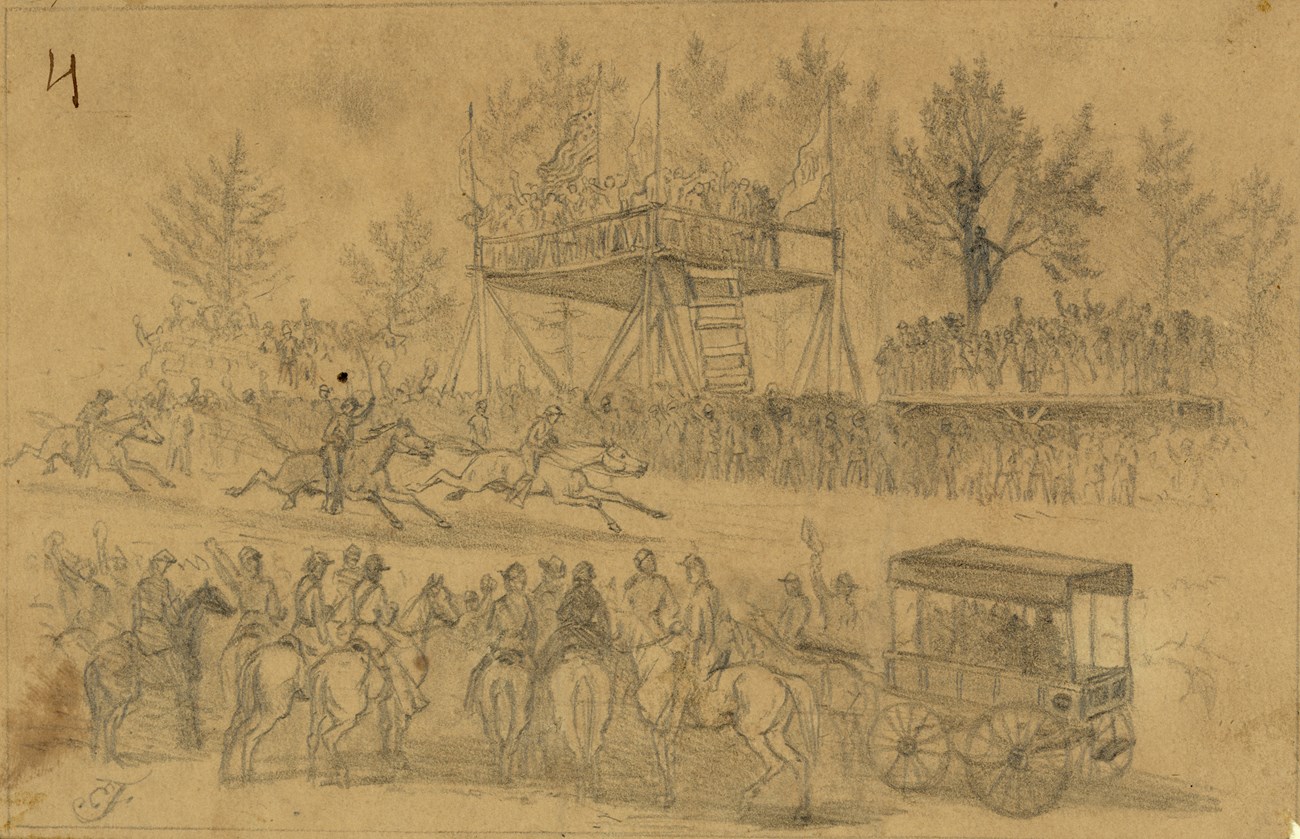This image depicts a detailed pencil sketch on a beige, oldish piece of paper, characterized by its orange or woody appearance. The paper is a horizontal rectangle, roughly twice as wide as it is tall. In the upper left-hand corner, there is a handwritten number four in ink. The sketch illustrates a bustling outdoor scene centered around a horse race. There are three horses racing along a central path, ridden by jockeys, and moving to the right at high speed. A diverse crowd of people surrounds this race, creating a sense of excitement and activity.

In the lower part of the image, a group of men in uniforms sit atop horses, and a horse-drawn cart is visible on the right-hand side. Above this scene, more men are engaged in the horse race. The background showcases a wooden, elevated platform with a ladder leading up to it, crowded with spectators. The platform is adorned with flags at each corner and features a prominent American flag in the center. Additionally, trees with more people standing among them are visible in the backdrop, further adding to the sense of a well-attended event. The sketch captures the lively atmosphere and detailed elements of a mid-19th-century horse race, including the energetic crowd, the racing horses, and the structured spectator areas.